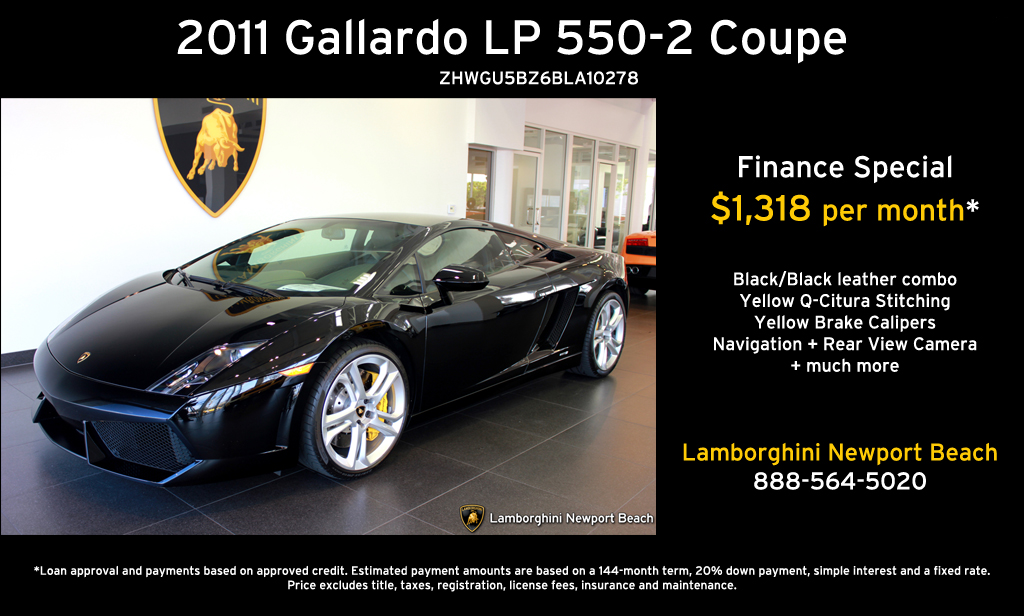The flyer is a sleek promotional ad for a 2011 Lamborghini Gallardo LP550-2 Coupe, featuring a luxurious black exterior with a matching black leather interior. Highlighting a finance special at $1,318 per month, the advertisement from Lamborghini Newport Beach boasts yellow Q-CITURA stitching, yellow brake calipers visible through the aerodynamic wheels, and advanced features such as navigation and a rearview camera. The dealership's contact number is 888-564-5020. The Lamborghini emblem is prominently displayed on a white wall next to the car, emphasizing the brand's prestigious appeal. The bottom of the flyer notes that loan approval and payment are based on approved credit, with additional details available in the small text.